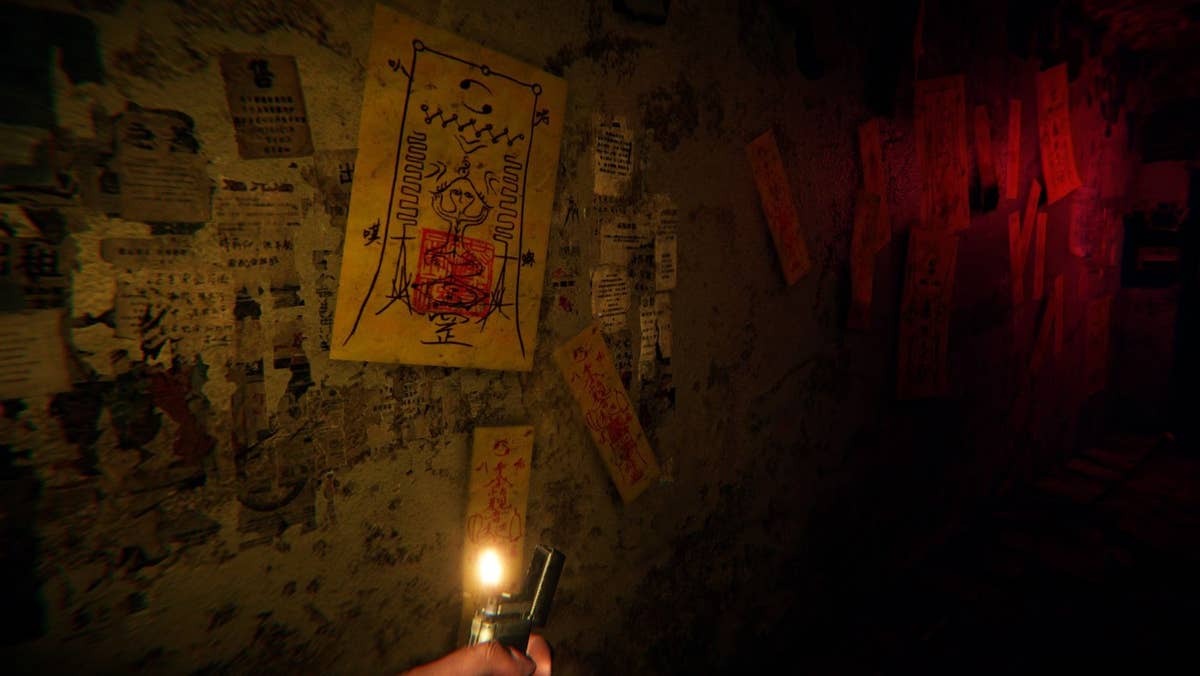The image is a horizontally-oriented, dark indoor scene that appears reminiscent of a cave or cavern. In the foreground at the bottom, there's a person's hand holding an older-style canister lighter that is lit, casting a small flame. The walls, which look like old, wood-paneled surfaces, are adorned with various items, including tan and brown posters featuring squiggly lines and patterns that resemble hieroglyphics. On the wall, there are also papers and possibly a child's drawing that appears red and extends to the top of its paper, though it’s partially obscured by the darkness. The right side of the wall is marked with rusty, red patches, enhancing the aged and somewhat eerie ambiance of the setting.